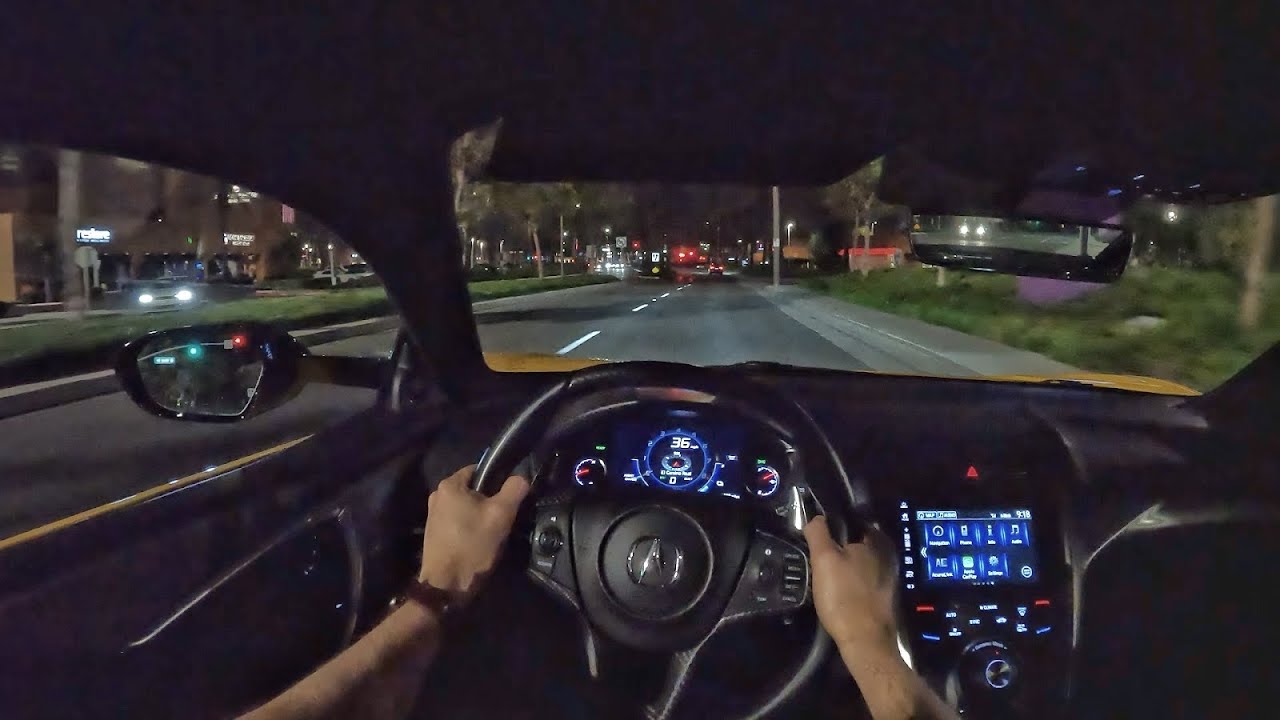This photograph captures a night-time scene from the perspective of a man driving an Acura down a city street. The driver, a white male, has his hands positioned at 9 and 3 o'clock on the illuminated steering wheel, which further highlights the lit dashboard, radio, heating, and air conditioning displays. The car, possibly a yellow taxi, moves along a two-way highway at 36 miles per hour. Through the vehicle's windows, one can observe a cityscape with buildings, street lights, trees, and cars on both sides of the street. Additionally, the side mirror reveals a green and red light, possibly indicating traffic or a vehicle in the driver's blind spot.